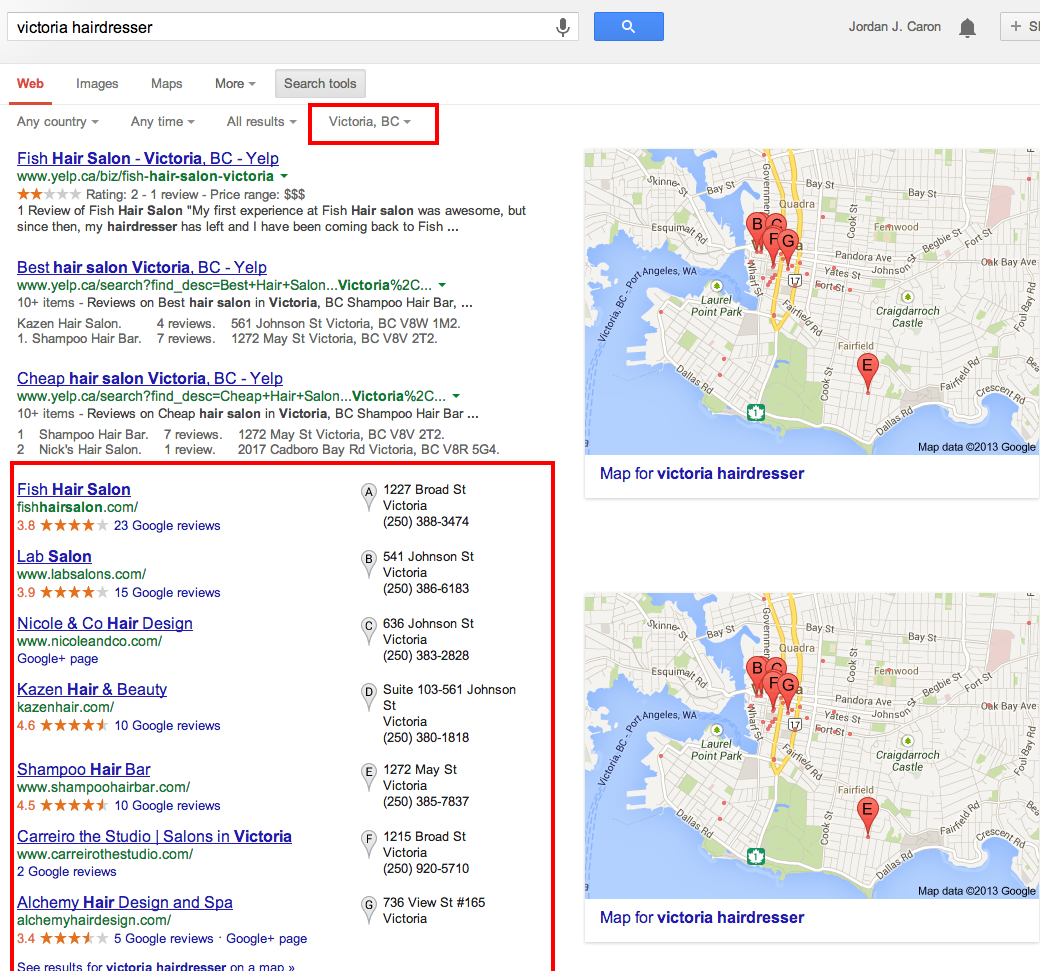The image depicts a large website interface, likely a search engine results page, focused on hairdressers in Victoria, British Columbia. At the top, there is a search bar containing the text "Victoria hairdresser," with a microphone icon and a blue box featuring a search icon next to it. The upper section of the page displays user profile names "Jordan J Karen" and an alert bell icon.

Below, a navigation menu shows tabs for "Web," "Images," "Maps," "More," and "Search tools," with "Web" highlighted in red. The search results include text suggesting popular queries like "fish hair salon Victoria BC," "best hair salon Victoria BC," and "cheap hair salon Victoria BC," which are all provided by Yelp.

To the right of these text results, there is a map marked with pins labeled B, C, F, G, and E, indicating the locations of different hair salons.

Further down the page, there is a red-bordered box listing various hair salons in Victoria: Fish Hair Salon, Lab Salon, Nicole and Company Hair Salon Design, Kaysen Hair and Beauty, Shampoo Hair Bar, Camero The Studio, and Alchemy Hair Design and Spa. Adjacent to this list is another map with red pins showing the precise locations of these establishments. The integration of the map alongside the detailed list helps users quickly identify and locate the salons in Victoria, BC.